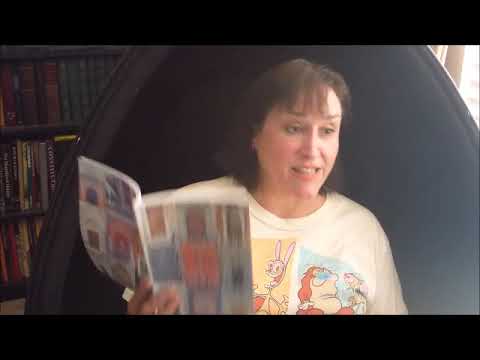A middle-aged white woman with medium to short, straight brown hair just above her shoulders, sits in a black, oval-shaped chair. She is wearing a white t-shirt adorned with colorful cartoon graphics, including what looks like a rabbit and a cartoon woman’s face with dark hair. In her right hand, she holds an open magazine or magazine-shaped book featuring a cover composed of a 3x3 grid of pastel-colored squares, although the cover is somewhat blurred. The woman is not looking at the book but gazes off to her left. Behind her, on the left side of the image, is a bookshelf with rows of books, and on the right side, sunlight streams through, illuminating the left side of her face.